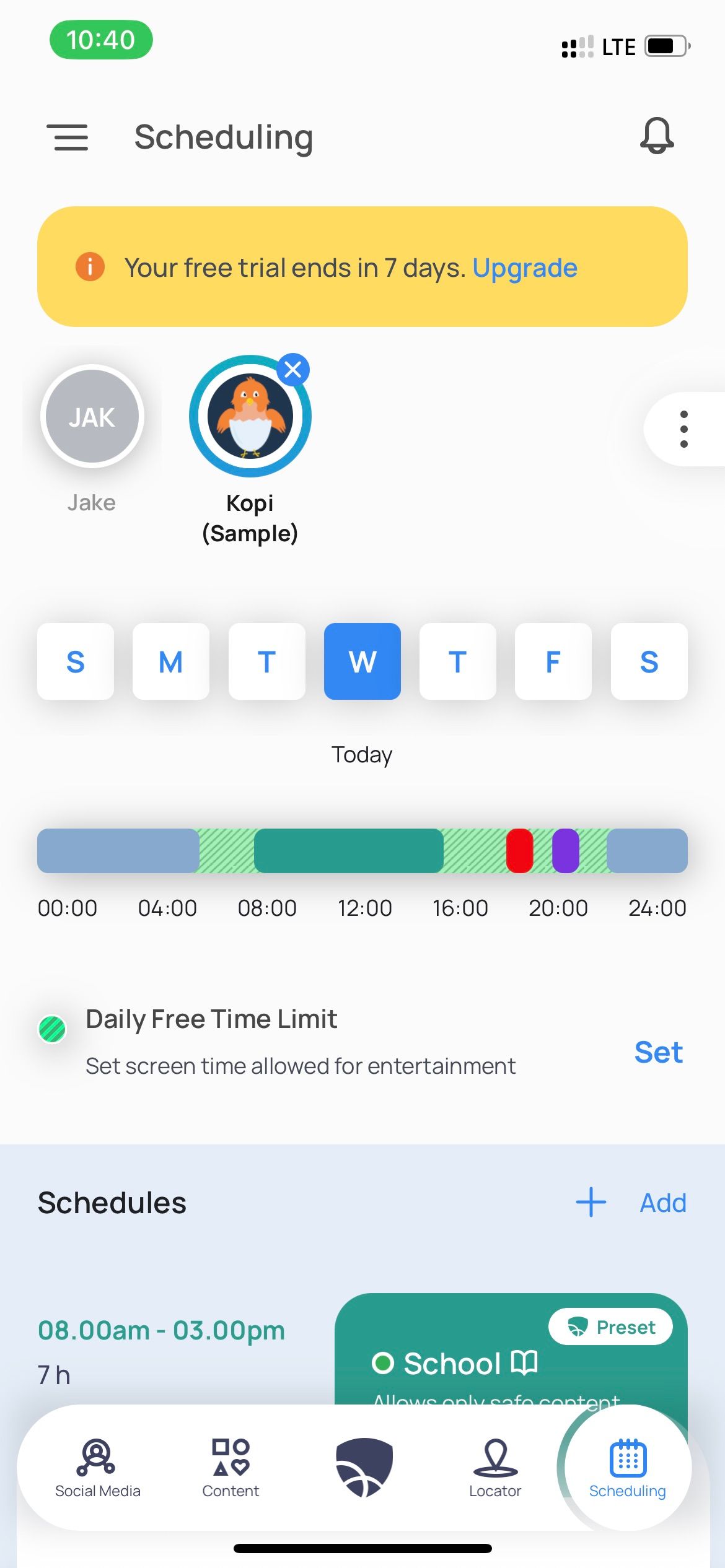This image is a mobile device screenshot showcasing a scheduling interface. At the very top of the screenshot, there is a scheduling section, flanked by a notification bell on the right and an additional button on the left. Below this section, there is a yellow bubble featuring an orange and white information icon, which informs the user that their free trial ends in seven days and includes a hyperlink to upgrade.

The background of the page is white, and it contains various round "story" symbols. One of these symbols is highlighted and labeled “copy or copay sample,” depicting a bird inside it with a blue ring around it. Another symbol, labeled "check and shake," is shown in gray and white.

Further down, the days of the week are displayed in tile format, with Wednesday being highlighted. Below the weekday tiles, there is a bar indicating a "daily free time limit." The screenshot also includes various schedule entries and several buttons related to the application's functionality at the bottom of the interface.